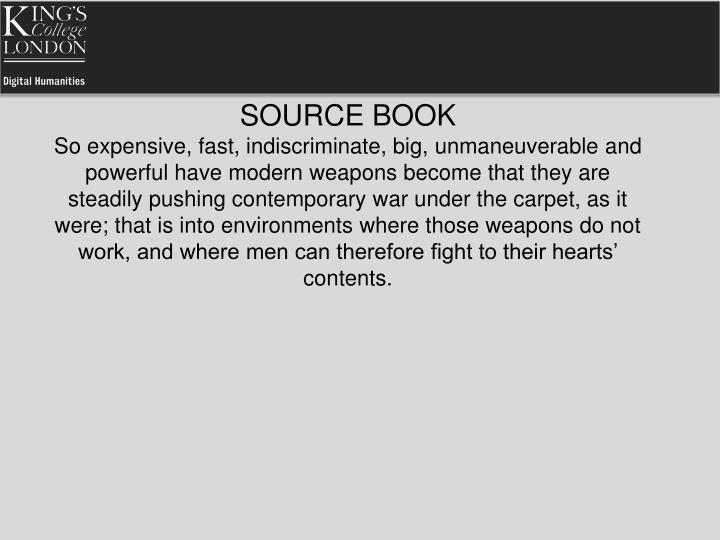The image is a slide with a black rectangular bar at the top and a gray background. In the upper left corner, the logo for King's College London Digital Humanities is displayed. The slide features black text in the center, reading: "Sourcebook. So expensive, fast, indiscriminate, big, unmaneuverable, and powerful have modern weapons become that they are steadily pushing contemporary war under the carpet as it were, that is, into environments where those weapons do not work and where men can therefore fight to their hearts' content." The design appears minimalistic, likely created on a platform such as PowerPoint, using a simple color scheme of black, white, and gray.